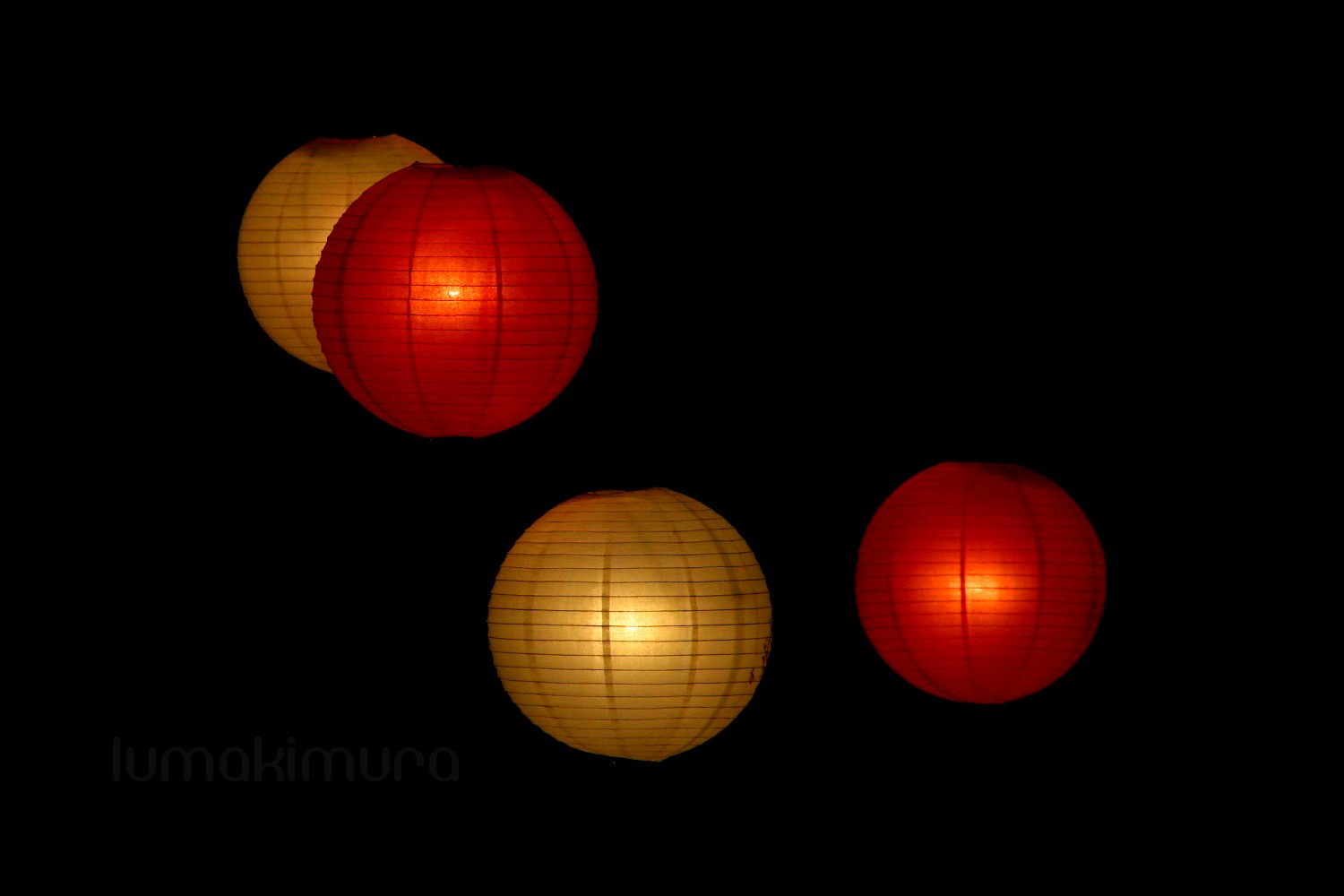This photograph captures a stunning nighttime display of four big, round Chinese lanterns set against a pitch-black background. The lanterns, which are used for lighting and decor rather than being released, emit a soft amber glow that beautifully illuminates their colors—two red and two yellow. The lanterns are arranged thoughtfully: in the top left corner, a yellow lantern is positioned beside a red one, while in the bottom center, another yellow lantern sits next to a red one on its right. Black stripes adorn each lantern, adding to their intricate design. Although the background provides no additional context, the subtle angling and even spacing of the lanterns suggest they might be strung up on a porch or similar structure, possibly attached to a pole. The absence of any other visual elements, such as stars or the moon, centers attention solely on these radiant lanterns, making them the focal point of this mesmerizing scene.